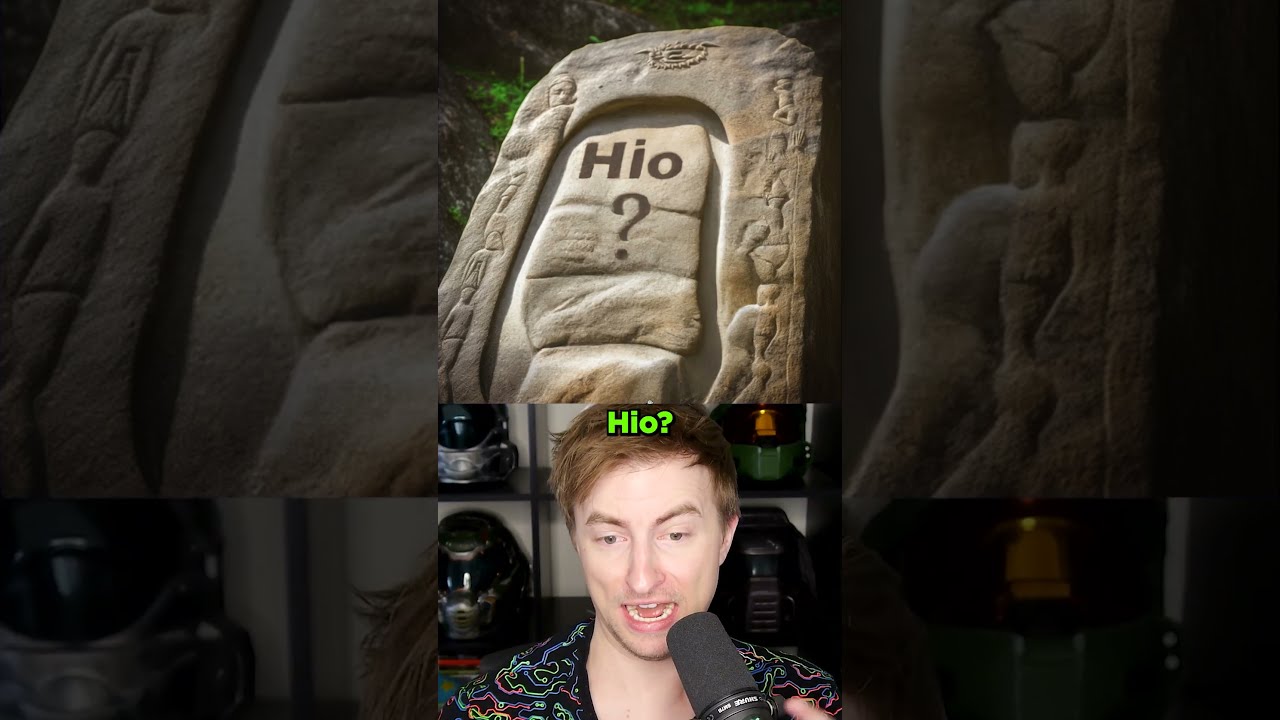In the image, there are two main sections arranged vertically, both with a darkened and zoomed-in version as the background. The bottom half features a close-up selfie of a young white man with light brown or orange hair, dressed in a patterned black shirt with green, purple, and yellow lines. He is speaking into a black microphone, facing slightly downwards with his mouth open, displaying his bottom row of teeth. Above him, in green letters, is the text "HIO?" Behind him, on black shelving, are various black items, including several helmets.

The top half of the image showcases an animated stone tablet with intricate carvings along its border. The tablet has engravings of different body types and a head, as well as a central section where the same green text "HIO?" appears, this time followed by a question mark on a second line. The stone tablet is overlaid with distinct graphical elements, giving it a detailed and textured appearance. The entire composition combines both photographs into a cohesive design, enhanced by the darkened and magnified background elements.